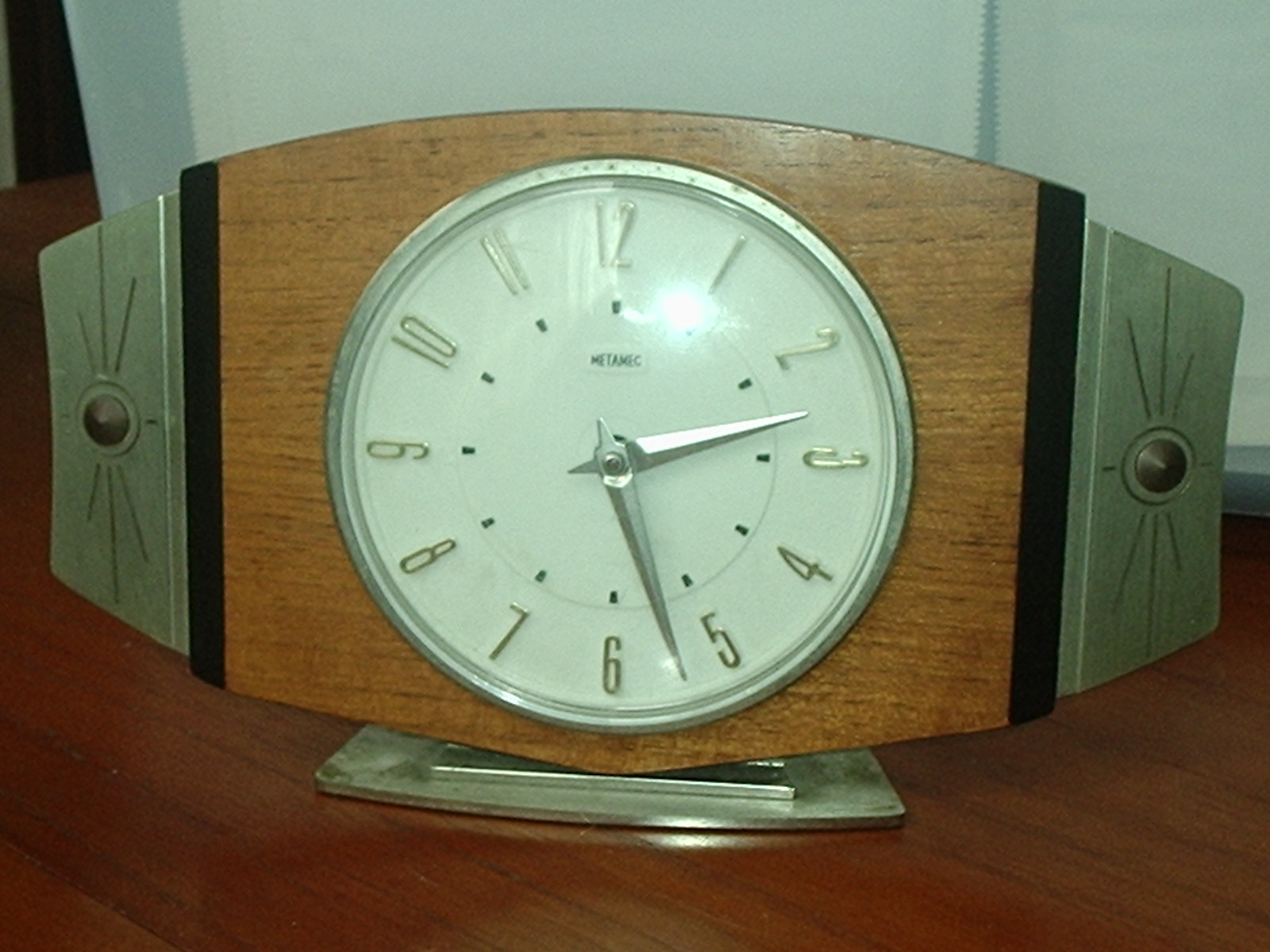A detailed caption for the image:

"An exquisite vintage desk clock, elegantly poised atop a dark oak table, radiates timeless charm. The clock boasts a pristine white face encircled by a polished silver lining, seamlessly attached to a sturdy oak wood frame. Below, a solid silver metal base provides balance and sophistication. Intricate silver attachments on the sides, featuring a star-like design with a circular center, enhance its antique allure. The clock face is adorned with sleek silver numerals and hands—featuring only the hour and minute hands—adding to its classic simplicity. This charming piece would be a perfect addition to a refined home office or a cozy living room."